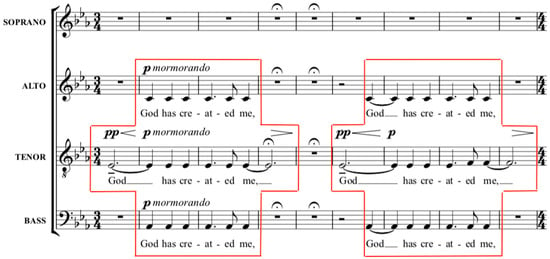The image features a detailed color infographic of a musical score on a solid white background. The score is divided into four staffs labeled on the left-hand side as Soprano, Alto, Tenor, and Bass. Each staff contains the same musical notes and lyrics, specifically the phrase "God has created me," sung twice per measure. The music is notated in 3/4 time, and visual markers such as red boxes highlight specific notes. The score includes various musical symbols like quarter notes, whole notes, rests, and other notation elements, all structured to show the distinct yet unified parts of the four vocal ranges.